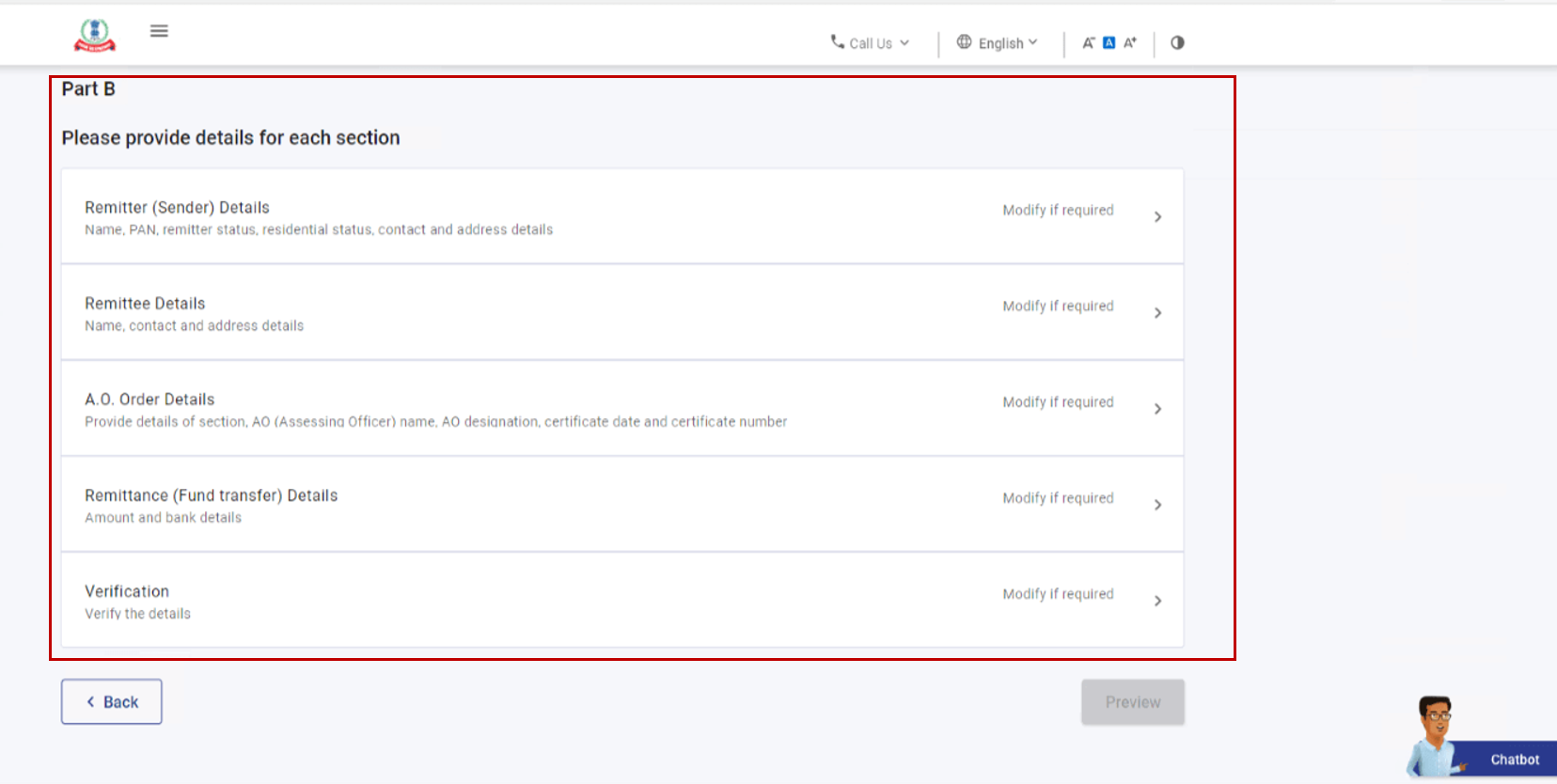This image is a detailed screenshot from a website interface. On the left side, partially obscured, is the website's logo. The logo consists of a primary circle in bluish color containing two smaller circles within it. Below the circles is an elegant red curve interspersed with text. 

Across the image is a prominently displayed red-outlined box with the heading "Part B." Inside this box, there is a clear instruction to "Please provide details for each section." 

The form is segmented into five key sections:
1. **Remitter (Sender) Details**: The section for entering the details of the sender.
2. **Remittee (Receiver) Details**: The section for entering the details of the recipient.
3. **AO Order Details**: Specific order information details related to the transfer.
4. **Remittance (Fund Transfer) Details**: This area captures the amount and bank details for the transaction.
5. **Verification**: A section dedicated to verifying the entered details.

Next to each of these sections on the right-hand side, there is a column labeled "Modify if required," where users can click to make changes.

Below this red-outlined box, there are two prominent buttons: a "Back" button to go to the previous page and a "Preview" button to review the details before submission.

Finally, in the bottom-right corner of the image is a small dark-complected cartoon man with glasses labeled "Chat Bot," indicating the presence of an interactive chat feature for user assistance.